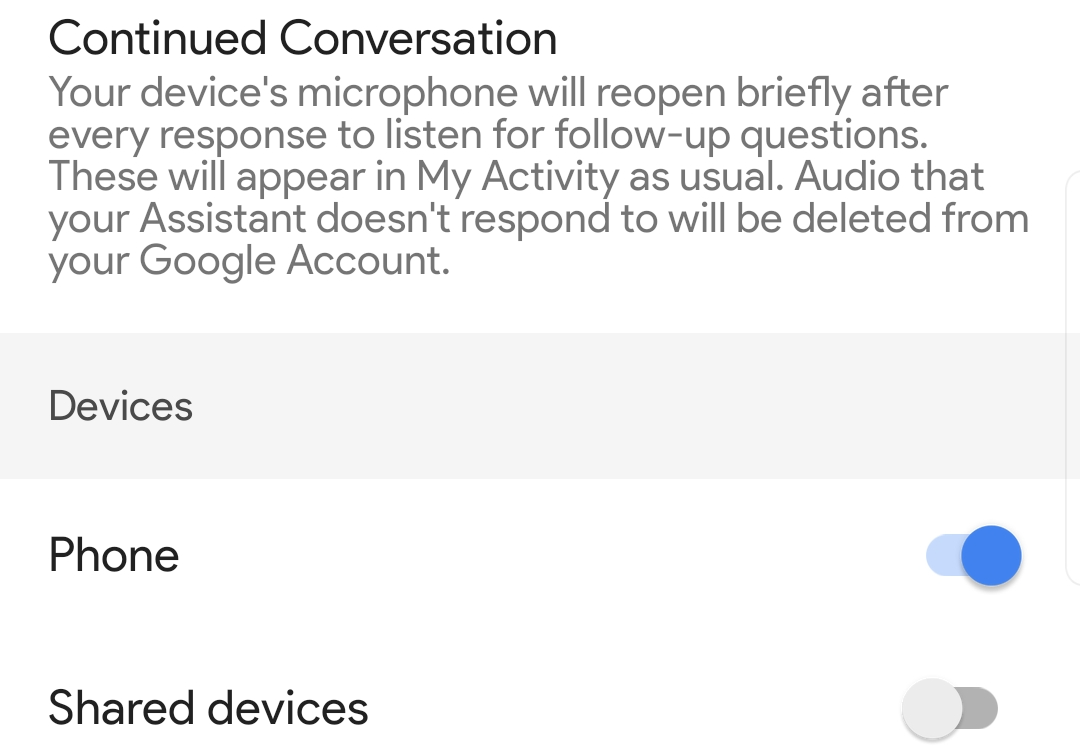The image features a structured interface on a predominantly white background. At the top, bold black text reads, "Your Continued Conversation." Below this, gray text states, "Your device's microphone will reopen briefly after every response to listen for follow-up questions. Questions will appear in My Activity as usual. Audio that your Assistant doesn't respond to will be deleted from your Google account."

Beneath this explanation, there is a light gray box with the word "Devices" aligned to the left. Under this section, the background remains white. To the left, black text labels "Phone," next to which is a toggle switch. This switch is blue with a blue circle, indicating it is turned on. 

Further down, another section labeled "Shared Devices" in black text appears on the left. Accompanying this label is another toggle bar to the right. This switch is gray with a gray circle, signifying it is turned off. 

Below these elements is a white, empty area with a barely noticeable vertical line running to the right of the previously described switch. The design is clean and minimalist, providing a clear visual hierarchy for the settings displayed.